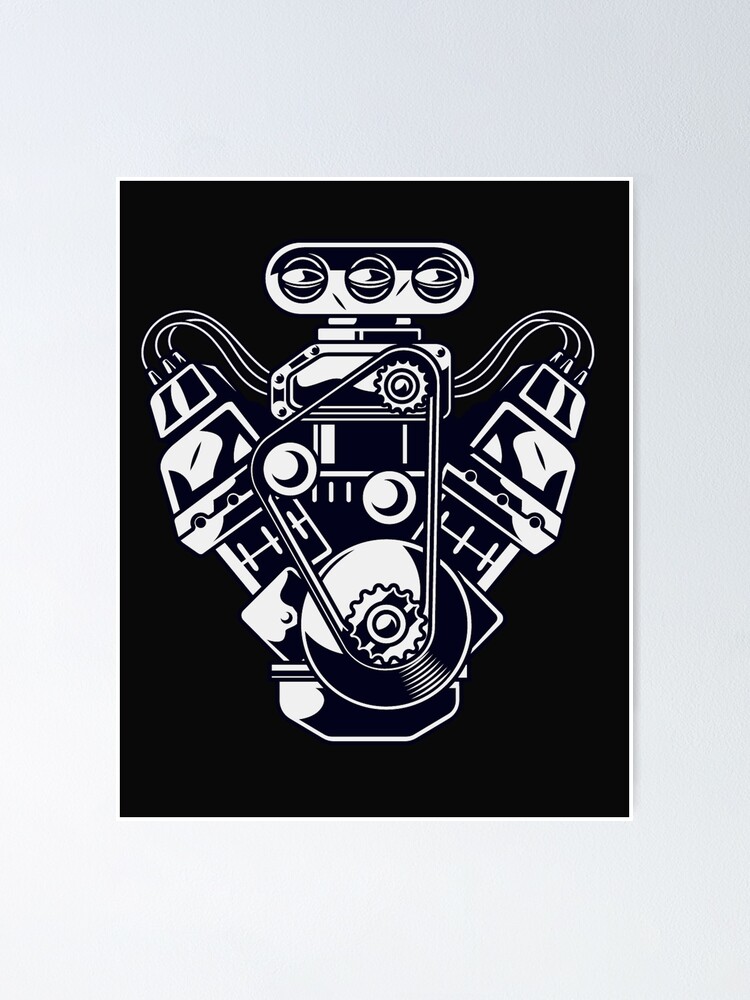The image is a detailed black and white drawing depicting the intricate inner workings of fantasy machinery. Set against a grayish-blue background with a solid black frame, the machinery features an array of cables, gears, and pulleys. At the top, there are three oval shapes resembling eyes or air intake valves. The central composition includes cables extending outward from a middle pulley, connecting to cylinders on either side. Above these cylinders, more cables converge towards an upper gear. The detailed machinery showcases various components such as a big wheel at the bottom, smaller nested wheels, and an interconnected band suggesting motion. There are also nuts, bolts, tubes, and a twisted knob, all adding to the complexity. It almost looks like the inner parts of a car engine or some sort of elaborate mechanical device.